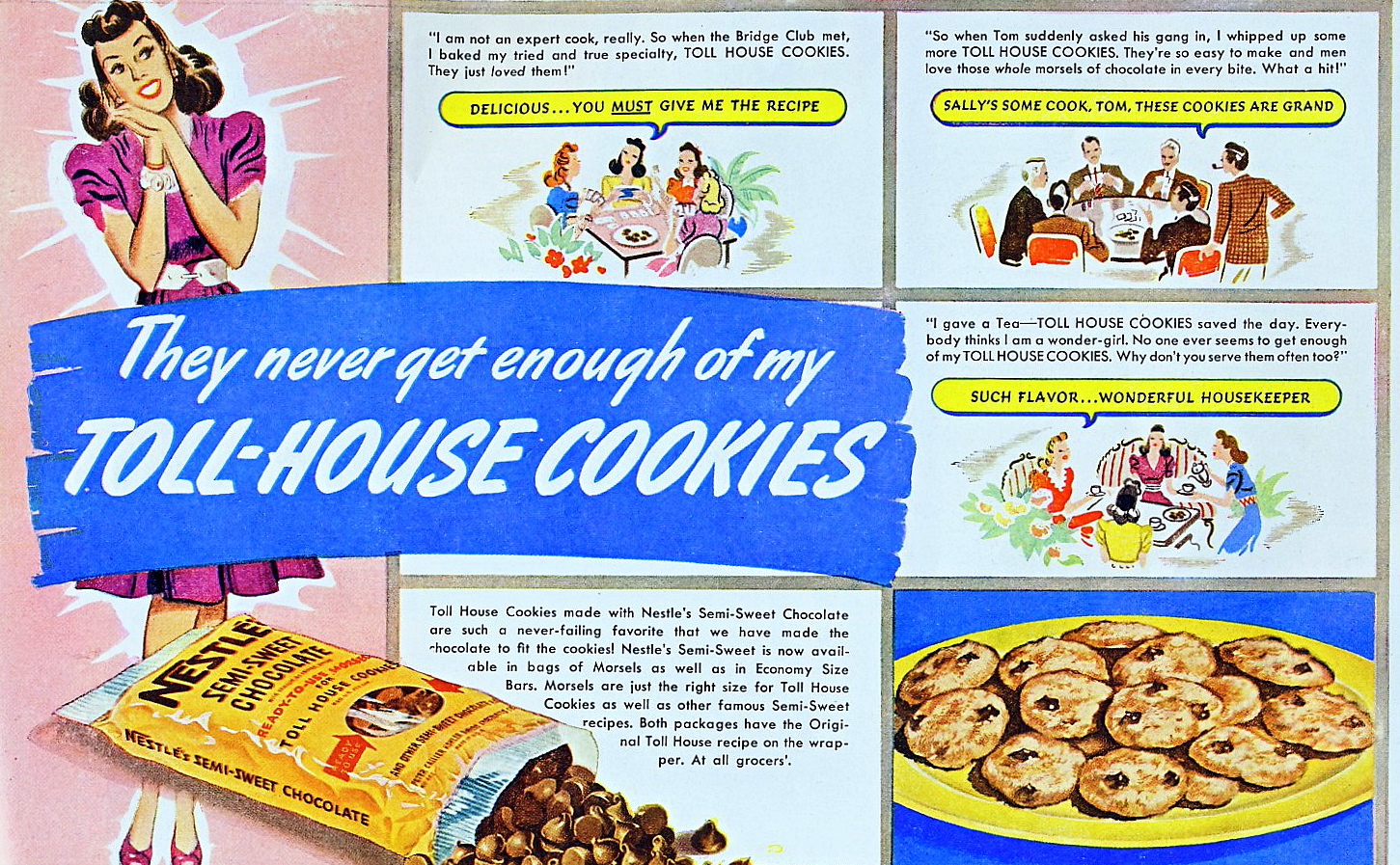This image is an old-fashioned advertisement from the 1950s for Nestle Toll House chocolate chip cookies, styled like a comic strip. At the center of the illustration is a brunette woman with a 1950s hairstyle, wearing a short-sleeved pink dress and white-pink high heels. She stands with her hands clasped under her chin in a thoughtful pose. A blue ribbon across the top reads, "They never get enough of my Toll House cookies." To her right, a series of comic panels feature dialogue that includes, "Delicious, you must give me the recipe," "Sally's some cook, Tom," "These cookies are grand," "Such flavor," and "Wonderful housekeeper." Additionally, there is a yellow bag of Nestle Toll House semi-sweet chocolate chips spilling out alongside a plate of freshly baked cookies, emphasizing their irresistible appeal. The ad communicates how these cookies can make any occasion special and highlights the ease of preparation and the joy they bring to everyone who tastes them.